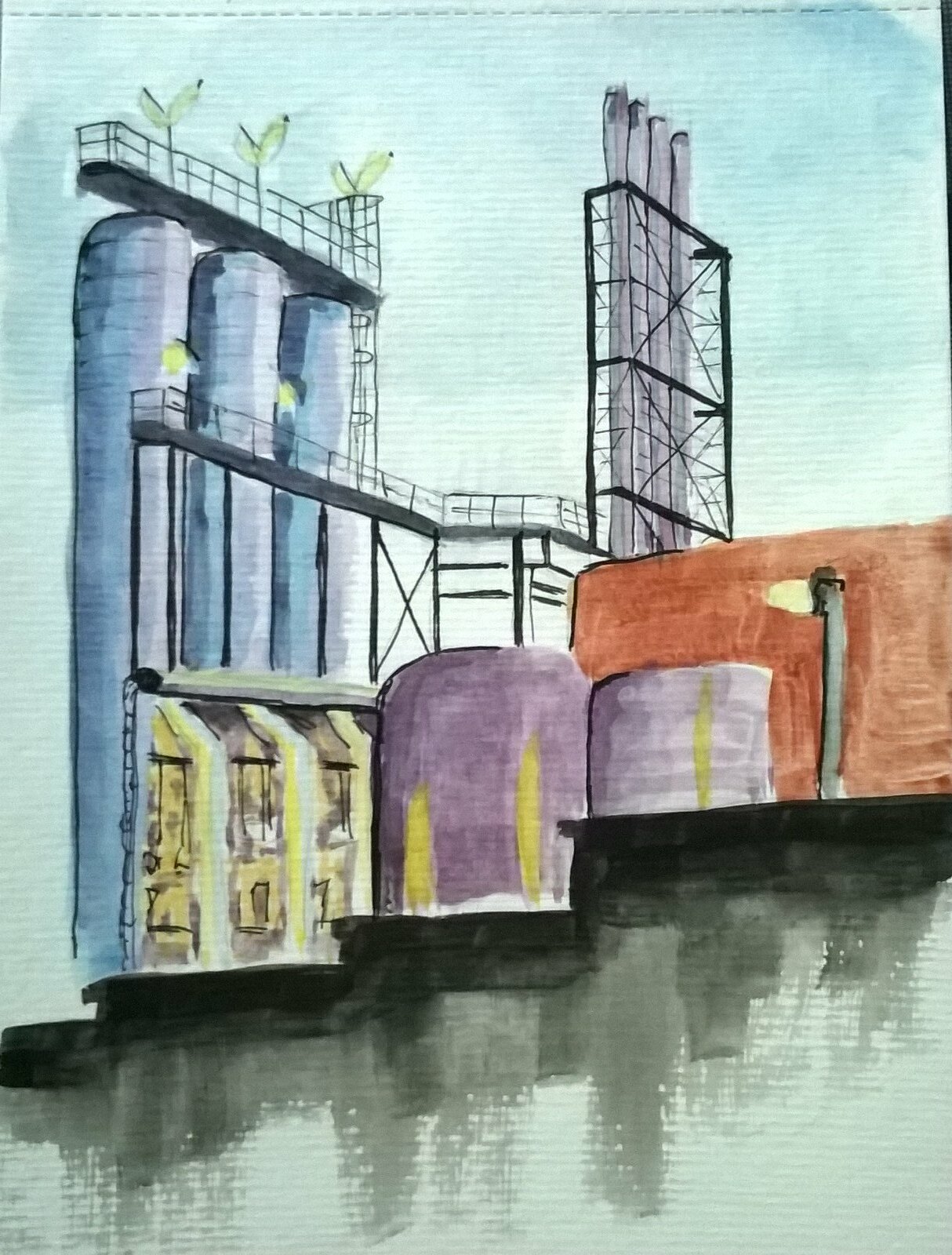This watercolor painting, rendered on linen paper, vividly captures the intricate structure of an oil refinery. The scene is dominated by several tall storage tanks and four towering smokestacks, encased in a network of scaffolding or cages, likely designed for maintenance access and structural support. Prominent catwalks connect various sections of the refinery, emphasizing its industrial complexity. In the foreground, large storage tanks are positioned close to the viewer's perspective, enhancing the sense of scale and depth. The painting reflects a serene, daytime setting, with clear skies and no emissions from the smokestacks, suggesting a moment of inactivity at the refinery.